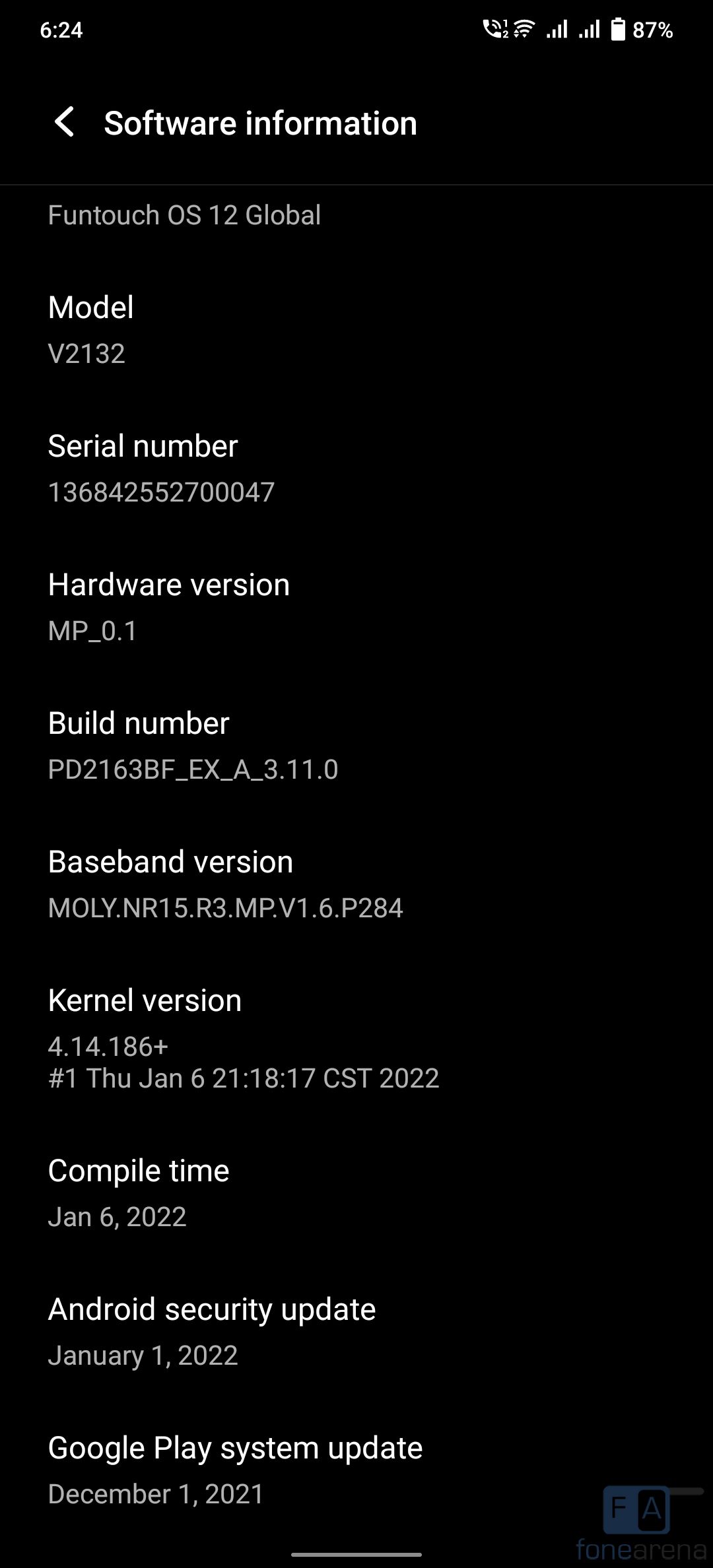A detailed on-screen display of a smartphone showcasing the device's software information. The battery indicator at the top right shows 87% life, adjacent to a strong network signal icon. The time displayed is 6:24. The screen is predominantly black with white and gray text elements. 

The top section prominently features "Software Information" with a left-pointing arrow. Below, it lists "FunTouch OS 1.2 Global" in white lettering. Subsequent sections provide detailed information about the phone's specifications: 

- Model: V2132
- Serial Number: a lengthy alphanumeric code
- Hardware Version: MP_0.1
- Build Number: another lengthy alphanumeric code
- Baseband Version: a series starting with letters
- Kernel Version: a numeric sequence alongside "Thursday, January 6" with a specific time
- Compile Time: January 6, 2022
- Android Security Update: January 1, 2022
- Google Play System Update: December 1, 2021

At the bottom, a light gray bar spans the width of the phone's screen, and a small icon featuring a half-blue, half-black box appears in the bottom right corner.